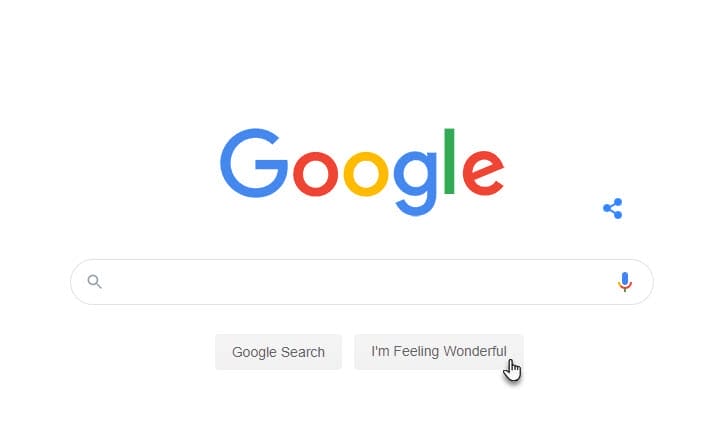This detailed caption describes a screenshot of the Google homepage:
 
The image is a screen capture of the Google website featuring its iconic multicolored logo comprising of a blue "G," a red "O," a gold "O," a blue "G," a green "L," and a red "E." Below the logo, there's a blue icon resembling a triangle. Further down, a gray search box is visible, containing a gray magnifying glass icon on the left side. To the right of the search box, there's a blue, red, and gold microphone icon. Underneath the search box, there are two rectangular buttons in gray with gray text: the left button reads "Google Search," and the right button reads "I'm Feeling Lucky," except for a nuanced tweak. A white mouse cursor, outlined in black, is hovering over the screen, contributing to the interactive feel of the image. The logo appears slightly pixelated, hinting at some image quality loss. The rest of the screen is free from any text or images, offering a clean, white background that highlights the elements described. The empty search box, clear design interfaces, and large font size give the impression that this is a zoomed-in view of the Google homepage.